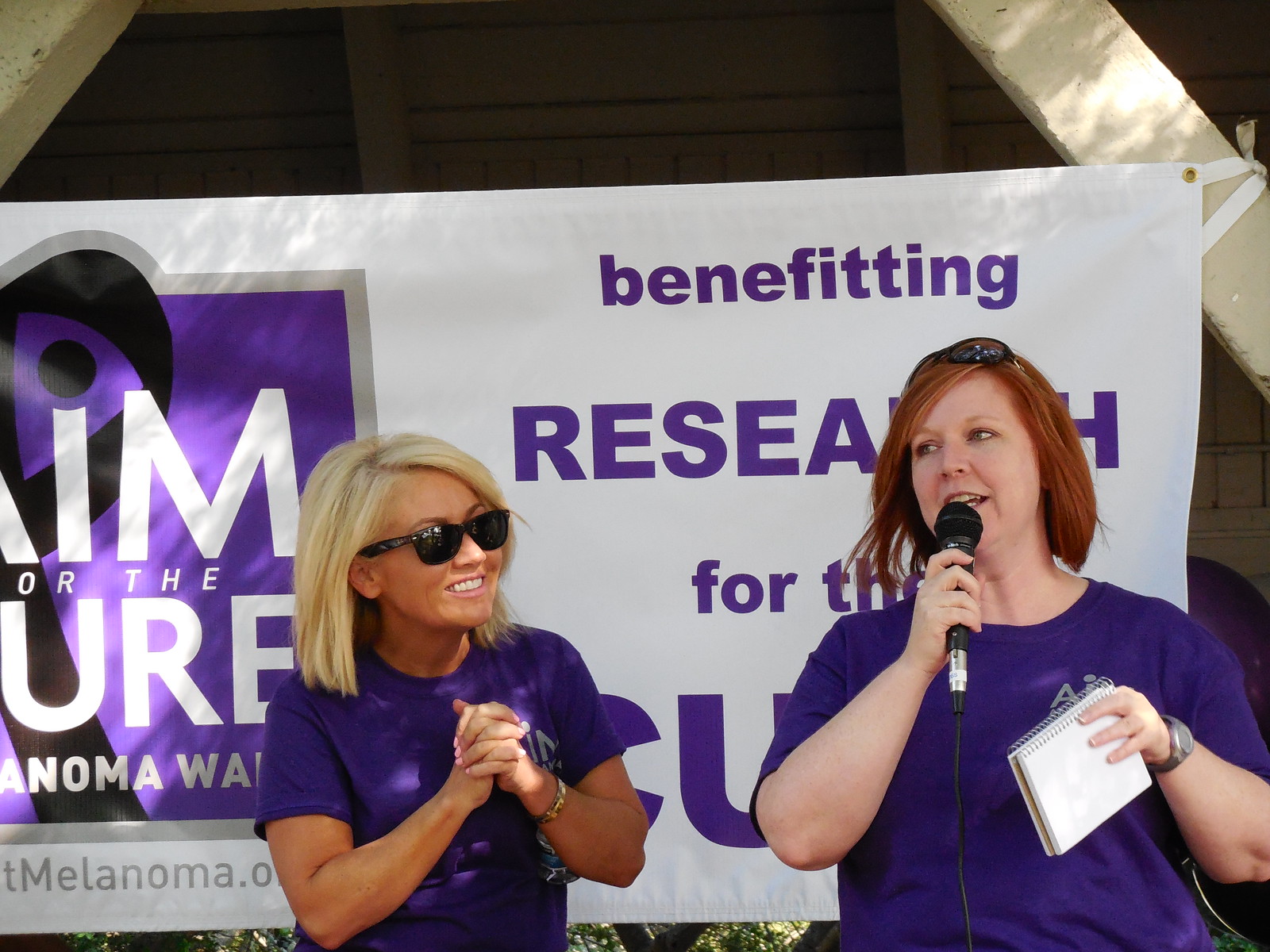In this image, two women are standing in front of a sign that suggests they are participating in a charitable event. Both women are wearing short-sleeved purple t-shirts. On the right, the red-haired woman is holding a wired microphone and has her sunglasses perched on top of her head. She has a small spiral notebook in her left hand and is wearing a watch on her left wrist. On the left, the blonde woman is wearing her sunglasses and has her hands clenched while smiling at the red-haired woman. She might also be wearing a wrist bracelet or a watch on her left wrist. The sign behind them is white with purple text, partially obscured by their positions, but the legible portion reads "Benefiting" and "Research for the." Additional visible text includes a website, likely "melanoma.org," indicating that the event is related to melanoma research. The overall scene suggests a fundraiser or awareness event, such as a race or walk, to support research for curing melanoma.